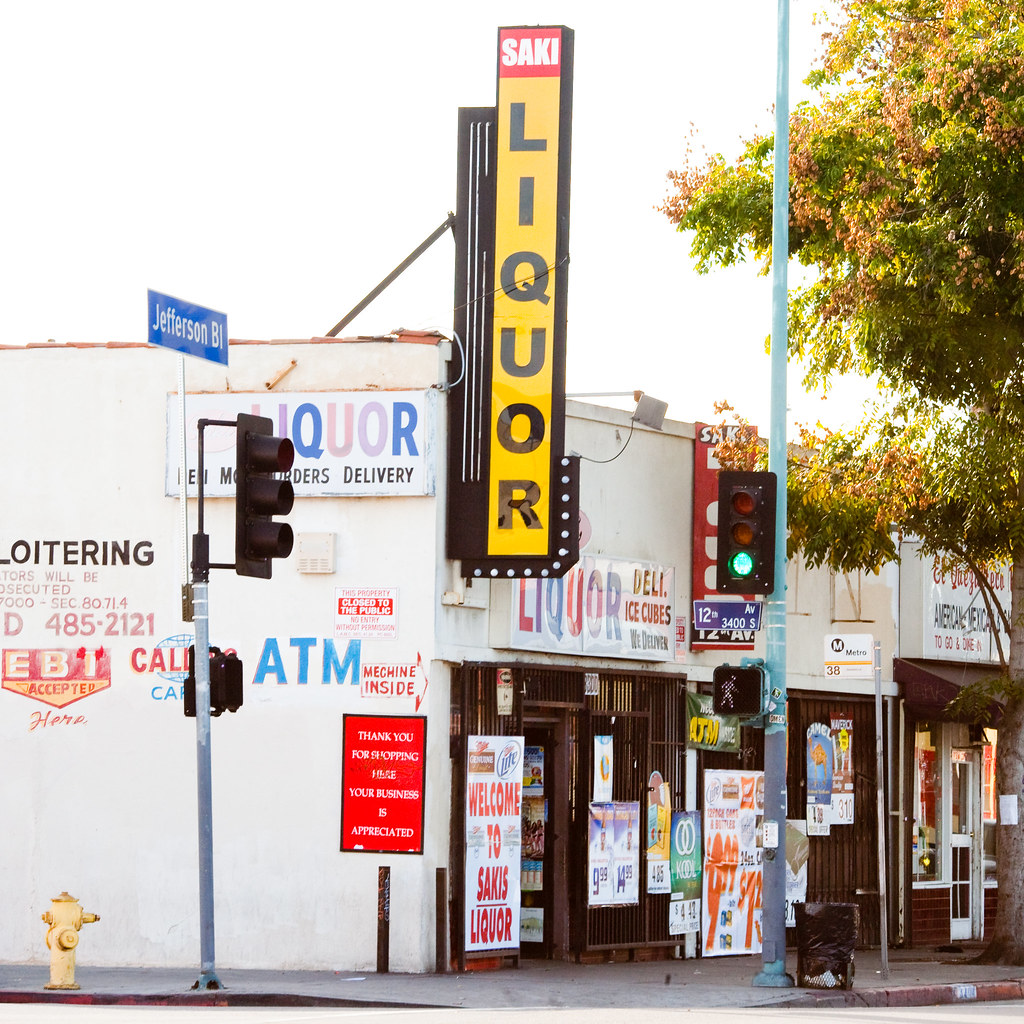The image captures the lively street corner of Jefferson B.L. and 12th Avenue, featuring the prominent Saki Liquor store. The storefront boasts vibrant signage with "Saki" in red with white lettering and "Liquor" on a yellow background with black lettering. Above the store, street signs mark the intersection. A green traffic light is visible, with another traffic light partially obscured. Various advertisements, including one for Cool cigarettes, decorate the store's front, which is secured by a metal gate, suggesting either early morning or a high-crime area. The side wall of the store has multiple notices, including "Loitering Prosecutors Will Be Prosecuted," "EBT Accepted," and "Thank you for shopping. Your business is appreciated." The description of the place extends to nearby storefronts, hinting at a busy urban setting.